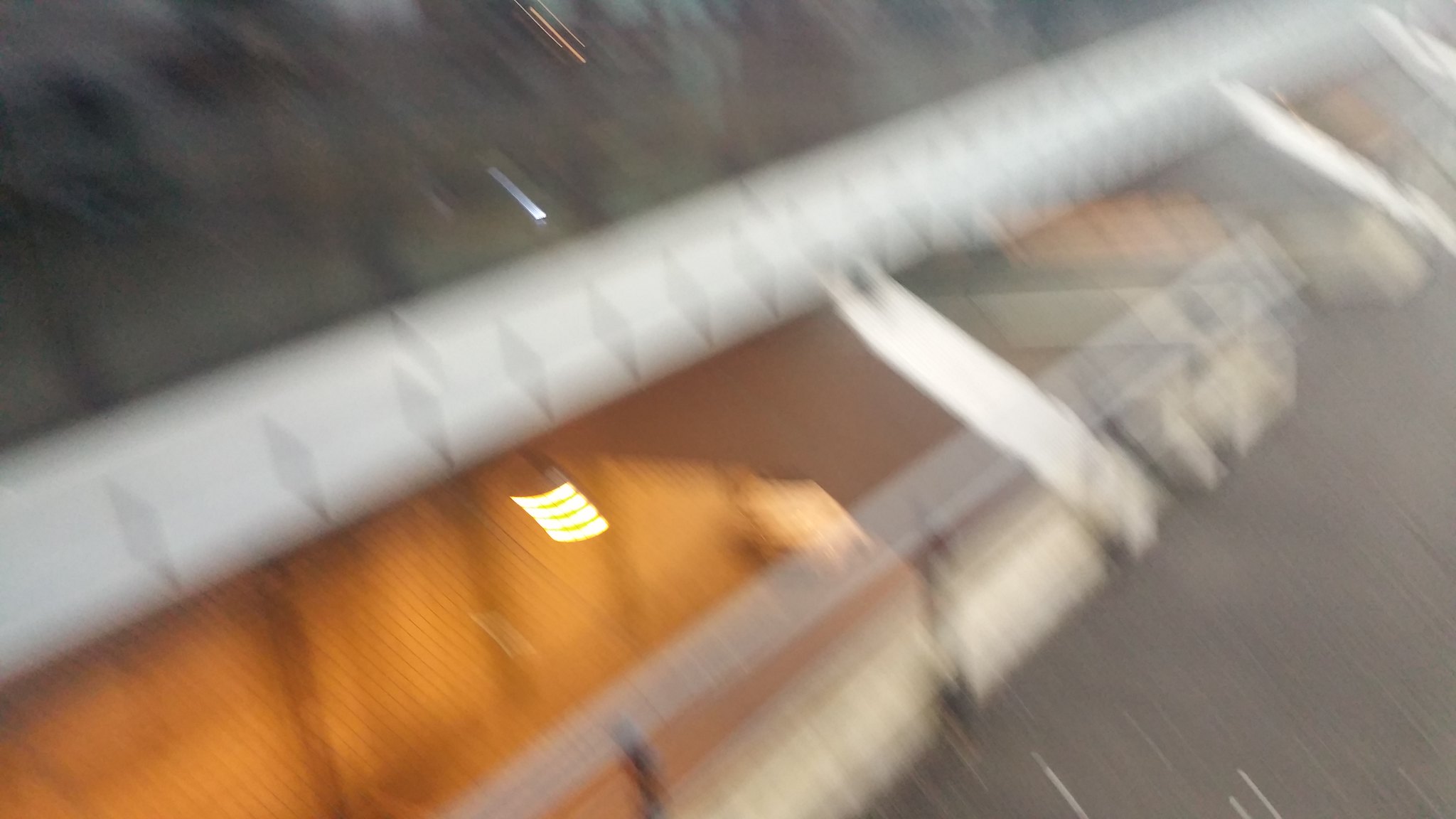The image is an extremely blurry and out-of-focus photograph, depicting an industrial site of sorts. The main feature in the image is a thick white pole, or railing, which extends diagonally from the bottom left corner to the top right corner of the picture. This railing is supported by several smaller white beams anchored to a possibly concrete or brown ground barrier. There is also a horizontal alignment of thin gray boards running across the bottom, lending an impression of a wooden bridge structure. A prominent feature is a silver barrier in a boxy shape, running across the image, encapsulating a large orange tent-like fabric structure. Above this, light illuminates the orange fabric with a golden hue, creating a subtle contrast against the overall grayish, gloomy background. The background in the top-left corner remains indistinct, composed of nondescript grayish colors, adding to the image's indistinct and somber ambience.